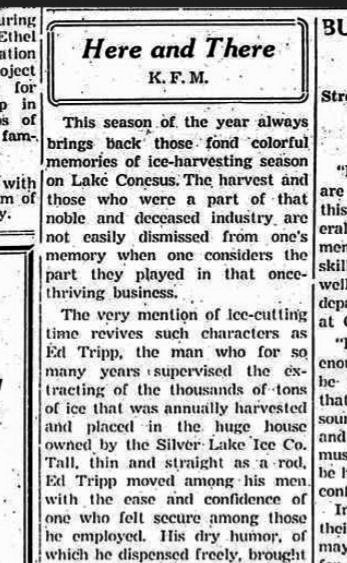The image is a close-up of a small section of a newspaper article that appears to be an old, somewhat degraded photocopy. The article is presented against a white background with black text and is divided into sections by vertical lines. At the top of the middle section, there is a small rectangular box containing the text "Here and There" followed by "KFM." Below this box, the article reads:

"This season of the year always brings back fond, colorful memories of the ice harvesting season on Lake Conesis. The harvest and those who were part of that noble and now defunct industry are not easily forgotten when considering the significant role they played in that once thriving business. The mere mention of ice cutting time brings to mind characters such as Ed Tripp. For many years, Ed Tripp supervised the extraction of thousands of tons of ice, which was annually harvested and stored in the massive ice house owned by the Silver Lake Ice Company. Tall, thin, and straight as a rod, Ed Tripp managed his men with ease and confidence, his dry humor freely dispensed." 

The text gets cut off at the bottom, leaving the final part incomplete. The photocopy shows additional text on the left and right edges that is cut off, and the overall quality of the image is poor, marked by black dots and a general sense of wear.